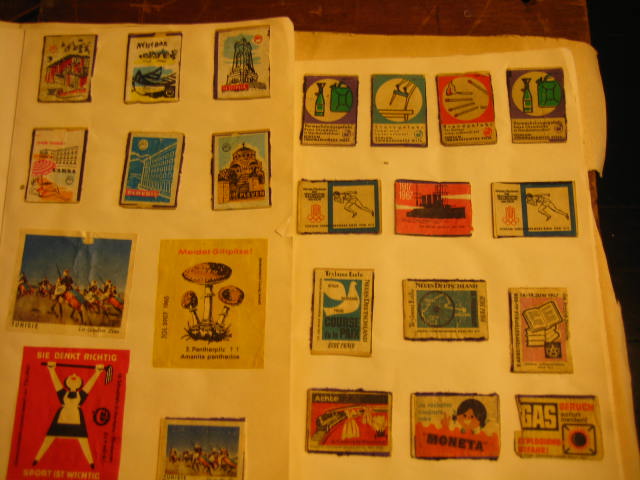The image depicts a warmly lit photograph of what appears to be a vintage postcard or stamp collection, though it's not entirely clear what the small pieces of paper are. The collection, which spans across two pages, features various aged graphics glued onto white pages, organized haphazardly rather than in a typical stamp collector’s meticulous manner. Each page contains a differing number of pieces: one with ten and the other with thirteen. The pieces come in various orientations (landscape and portrait) and sizes. Notable images include a stone tower, a mushroom, a bottle with a funnel next to a gasoline can, and a woman holding a mop above her head. Some pieces have text like "Monita" and "gas," adding to the vintage and possibly eclectic nature of the collection. The collection exudes an aura of nostalgia and antiquity.